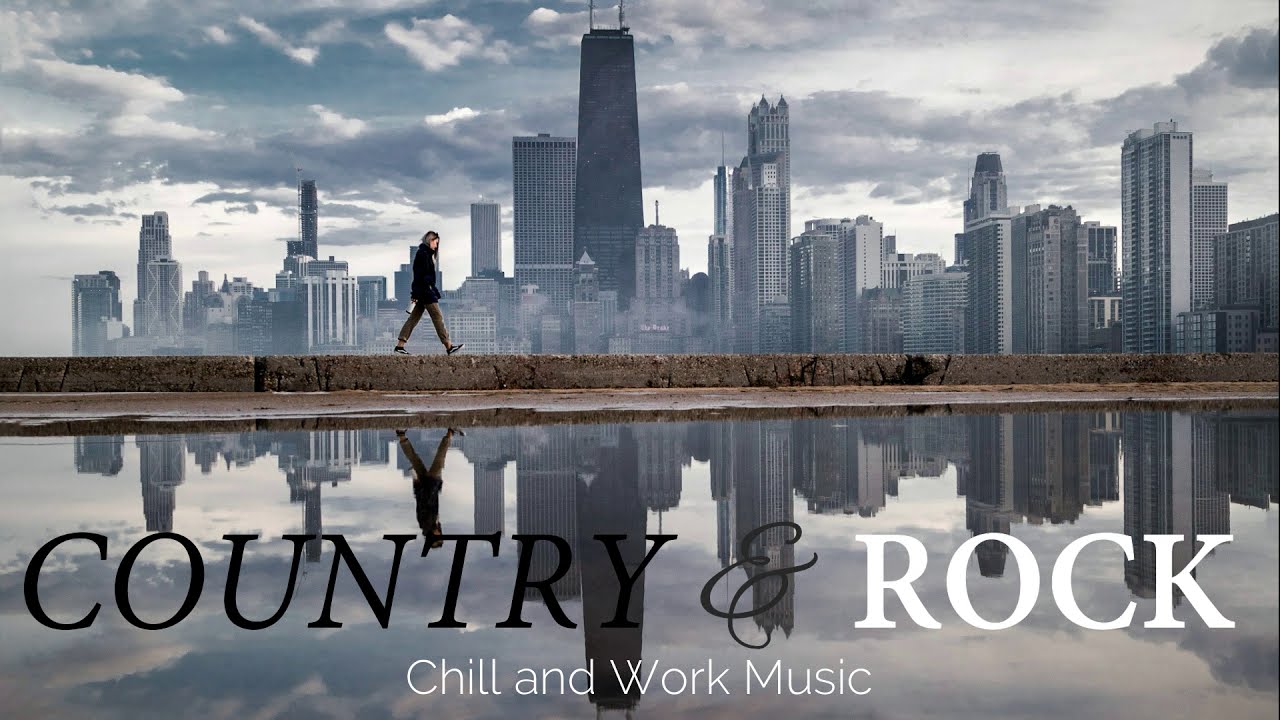The image is an advertisement for music, featuring a white woman with straight blonde hair walking on a brown stone or concrete pathway. She takes long strides while holding a water bottle. She's dressed in khaki or brown pants and a black jacket. The setting is a cloudy day, with a city skyline of gray and black toned skyscrapers in the background. At the bottom of the image is a body of water, reflecting both the cityscape and the woman. Overlaying the image are the words "country and rock, chill and work music" in black and white text.